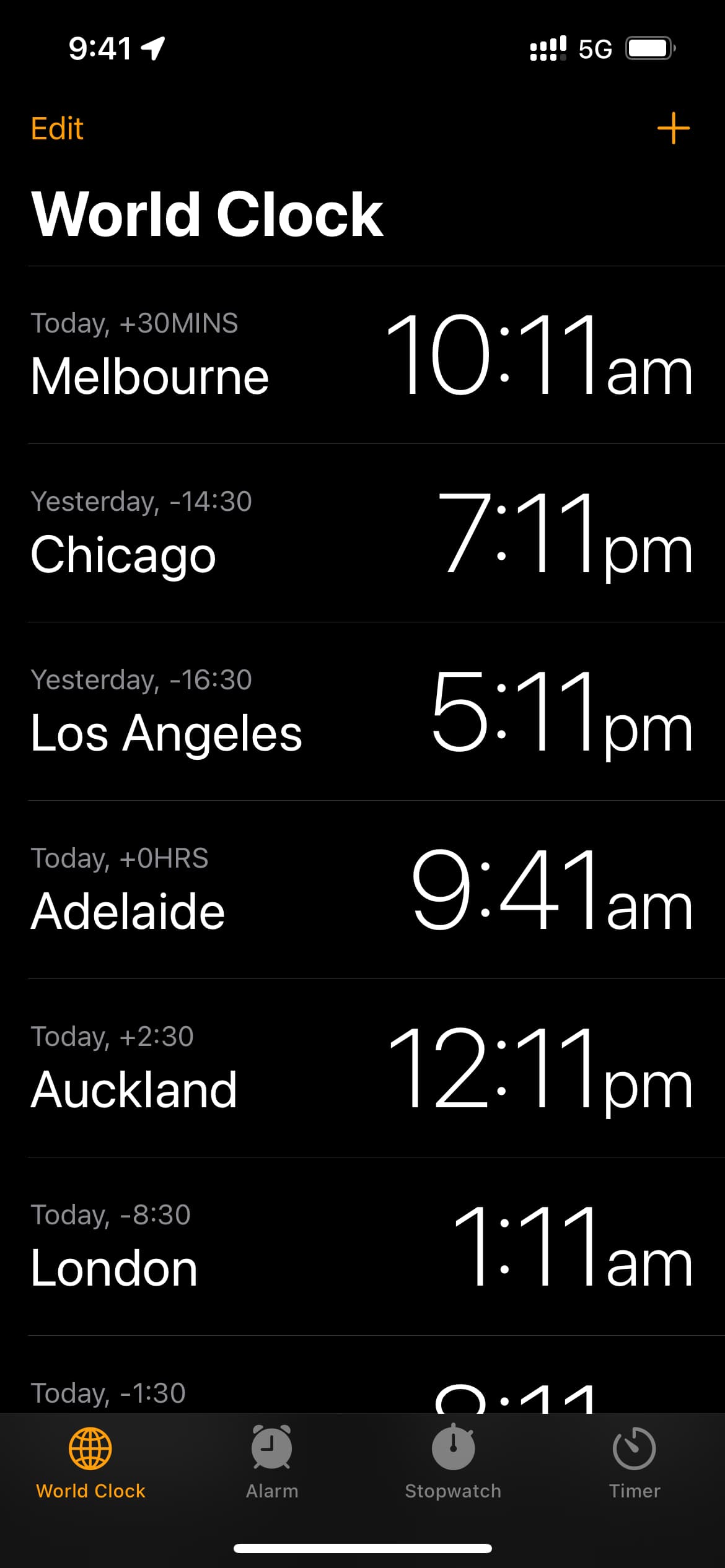The image features a black background with multiple UI elements displayed on it. In the top left corner, the time is shown as "9:41." The top right corner displays signal strength, indicating "5G," and a battery icon, showing around "90% battery." Below this, on the left side, there is an orange "Edit" button, and on the right side, a prominent orange "+" sign. 

In large white letters below the "Edit" button, the text "World Clock" is displayed. Underneath that, the screen lists various cities and their corresponding times and dates. 

- "Today +30 minutes, Melbourne: 10:11 a.m."
- "Yesterday -14 hours 30 minutes, Chicago: 7:11 p.m."
- "Yesterday -16 hours 30 minutes, Los Angeles: 5:11 p.m."
- "Today +0 hours, Adelaide: 9:41 a.m."
- "Today +2 hours 30 minutes, Auckland: 12:11 p.m."
- "Today -8 hours 30 minutes, London: 1:11 a.m."

Under this information, an orange globe icon is displayed with the text "World Clock" beneath it.

Overall, the image appears to be a snapshot of a mobile application's world clock feature, highlighting the current times in various global cities.